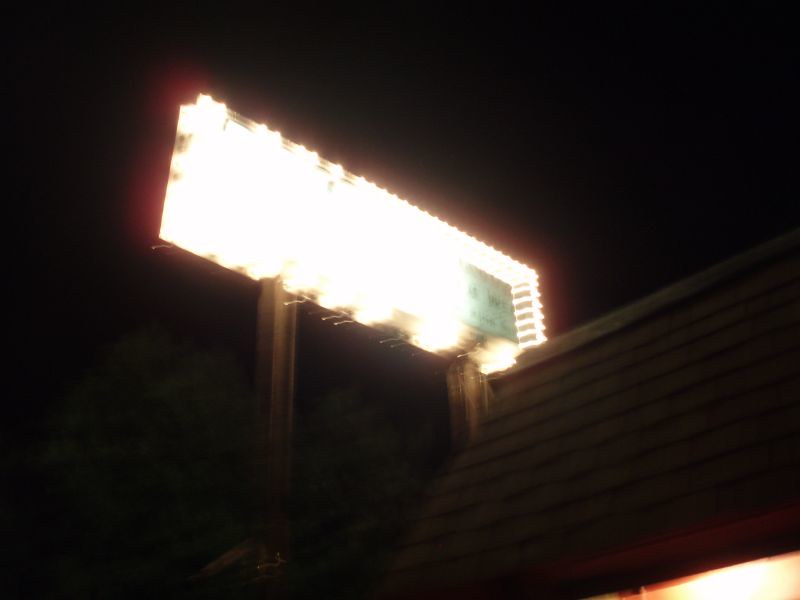In this nighttime photograph, the primary feature is a large, fully illuminated billboard that dominates the center of the image. The billboard, mounted on two sturdy stands, emits a bright light that obscures most of its content, save for a small, greenish-teal square with indistinct lettering. Surrounding the yellow lights that light up the billboard, a reddish glow adds a dramatic effect. The photograph, taken from a ground-level perspective, creates the impression of looking up at the towering billboard, underscoring its imposing presence. To the bottom right of the image, a steeply pitched roof leads up to about the midpoint of the frame, with some recessed lighting indicating part of a nearby structure. The rest of the image is enveloped in darkness, making the brightly lit billboard starkly stand out against the black night sky. The overall scene appears blurry, adding an eerie and mysterious quality to the photograph.